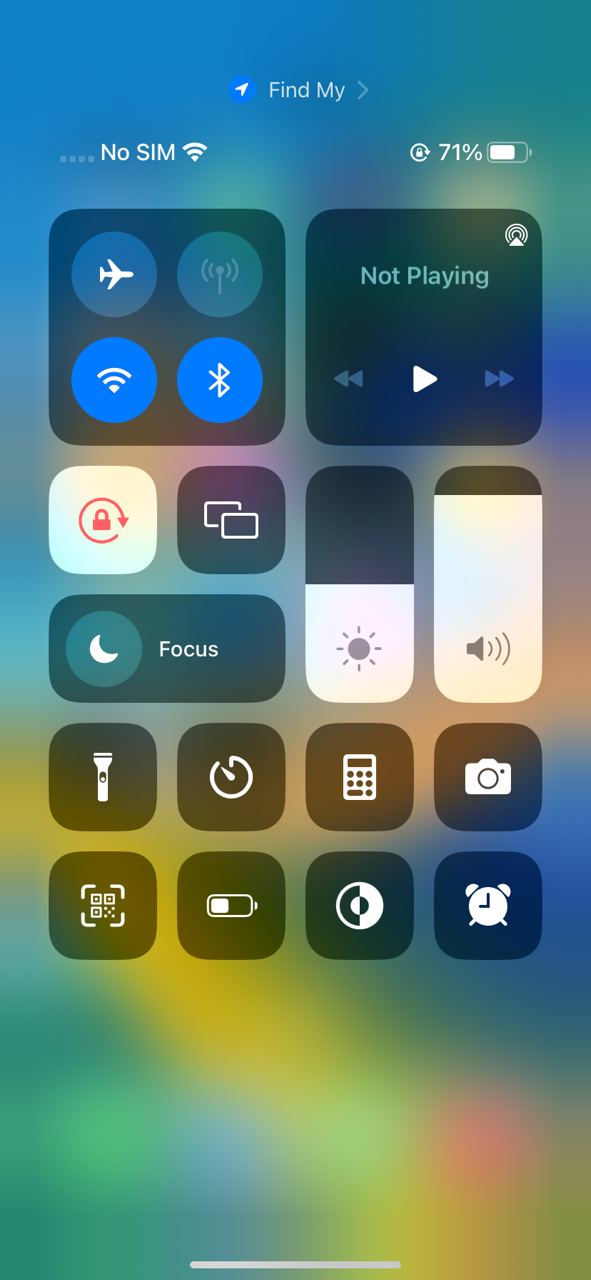The image is a screenshot from a cell phone, displayed in a vertical rectangular format. The screen features the "Find My" app prominently at the top, with the "No SIM" notification slightly lower and to the left. Next to these icons is a Wi-Fi symbol and a battery percentage indicator showing 71%, accompanied by a battery icon. 

The screen itself is the settings interface, highlighting various controls and tools. Notable features include the Airplane Mode icon, denoted by a small airplane, and the Wi-Fi button. There is also a media control widget labeled "Not Playing," equipped with play, fast forward, and rewind buttons. 

Further down, you can see the brightness adjustment slider set at about halfway, and the volume slider which is positioned quite high. Additional icons for utilities such as the flashlight, calculator, camera, and clock are present. In the background behind these buttons, there's a blurry, colorful display composed of yellow, green, and blue hues, giving the image a vibrant appearance.